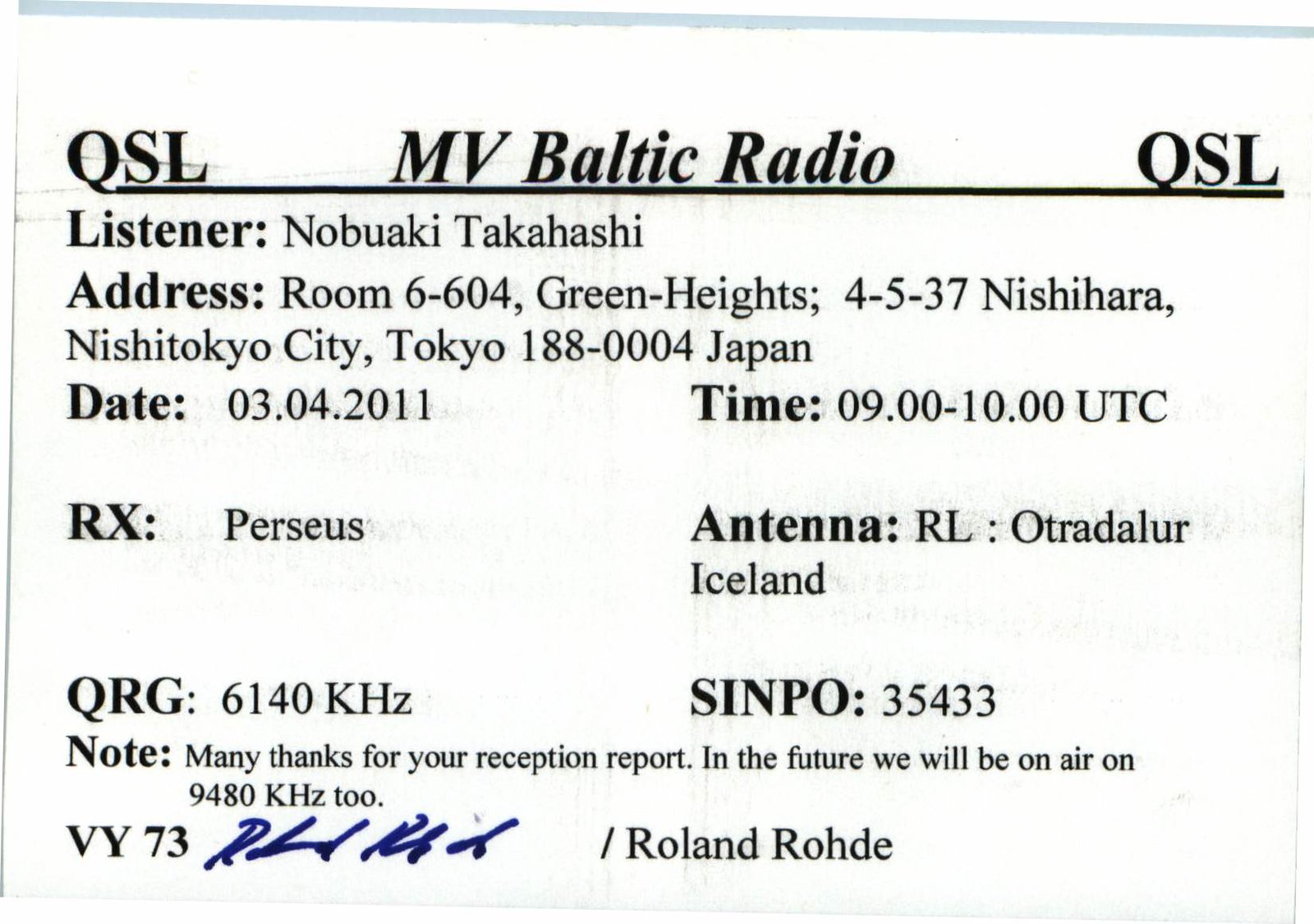The image is a scan of a printed QSL card with a white background and black text. At the top center, in large bold font, it reads "MV Baltic Radio," flanked by "QSL" in the top corners. Below this is a horizontal line, separating the header from the detailed information below.

On the left side, the bold word "listener" leads into the name Nobuaki Takahashi, followed by his address: Room 604, Green Heights, 4537 Nishihara, Nishitokyo City, Tokyo, 188004, Japan. Adjacent to this on the right is a section with the bolded word "date," showing 03-04-2011, and the bolded word "time," displaying 09-10-UTC.

Further down on the left, "RX" is bolded with "Perseus" in unbolded text beside it. Directly opposite this, on the right, "antenna" is bolded with "RL Otradalor Iceland" next to it in regular font. Below this, "QRG" is bolded with "6140KHZ" next to it, and to the right, "SINPO" is bolded with "35433."

Towards the bottom left, "note" is bolded, stating, "Many thanks for your reception report. In the future, we will be on air on 9480KHZ2." Below this, "VY73" appears next to a blue signature, likely made with a marker or pen, signed by Roland Rod.